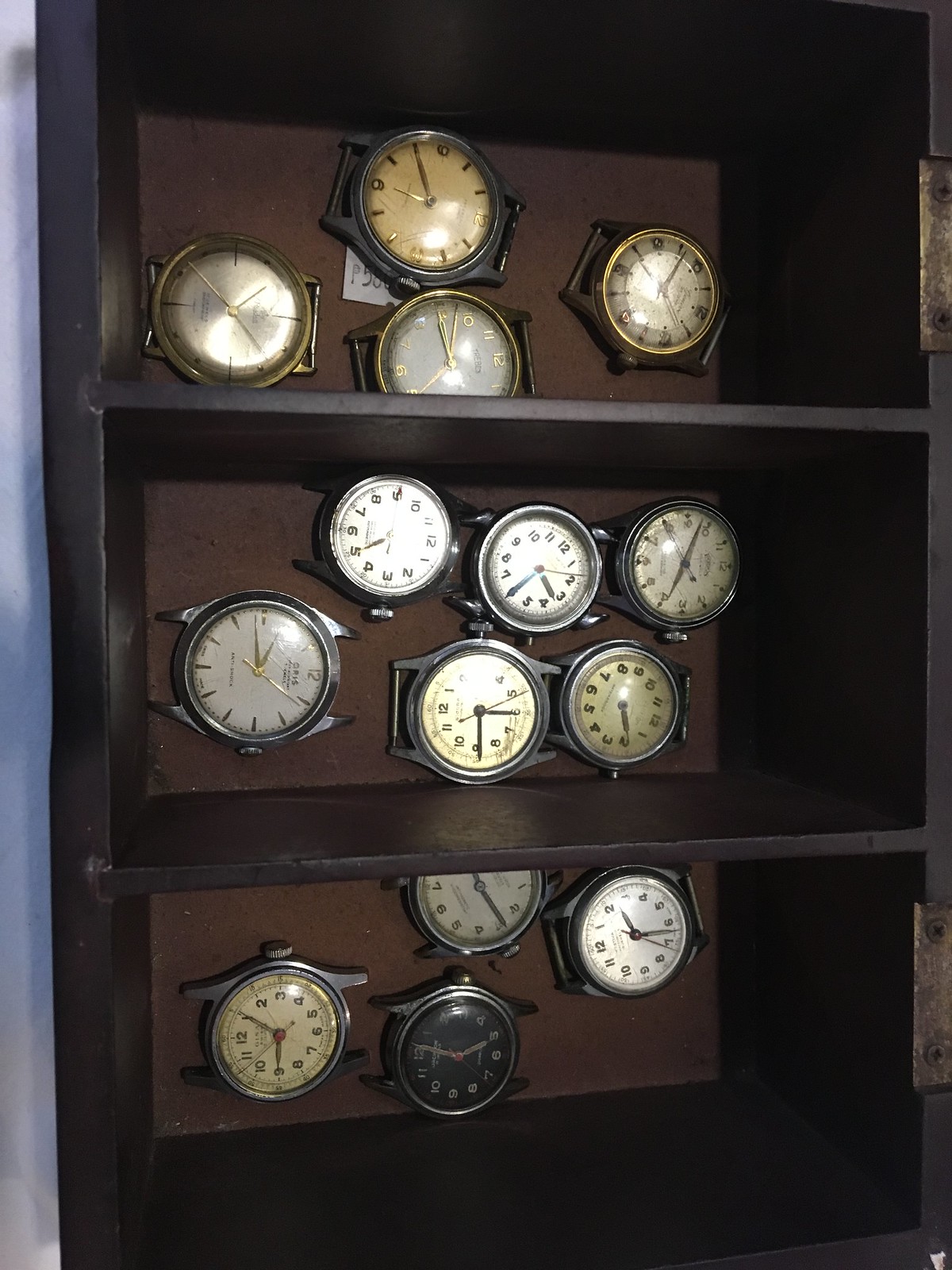The photograph depicts a dark brown wooden box with three shelves, possibly once part of an old jewelry box, given its hinges on the right-hand side. Each shelf contains an array of watch faces, notable for their antique appearance. 

In the top compartment, there are four watch faces, three of which feature a gold rim, while one has a silver rim. Among these, three have Roman numeral markings, and one displays regular numbers. The middle shelf holds six watch faces, all predominantly white except for two that are yellow. Some faces display numbers, while others have lines indicating the hours. The bottom shelf contains four watch faces with a mix of yellowish, black, white, and green colors. They all lack bands and show only the round metal faces with adjustment knobs. Some watches have numerical markings, contributing to their varied, aged aesthetic.